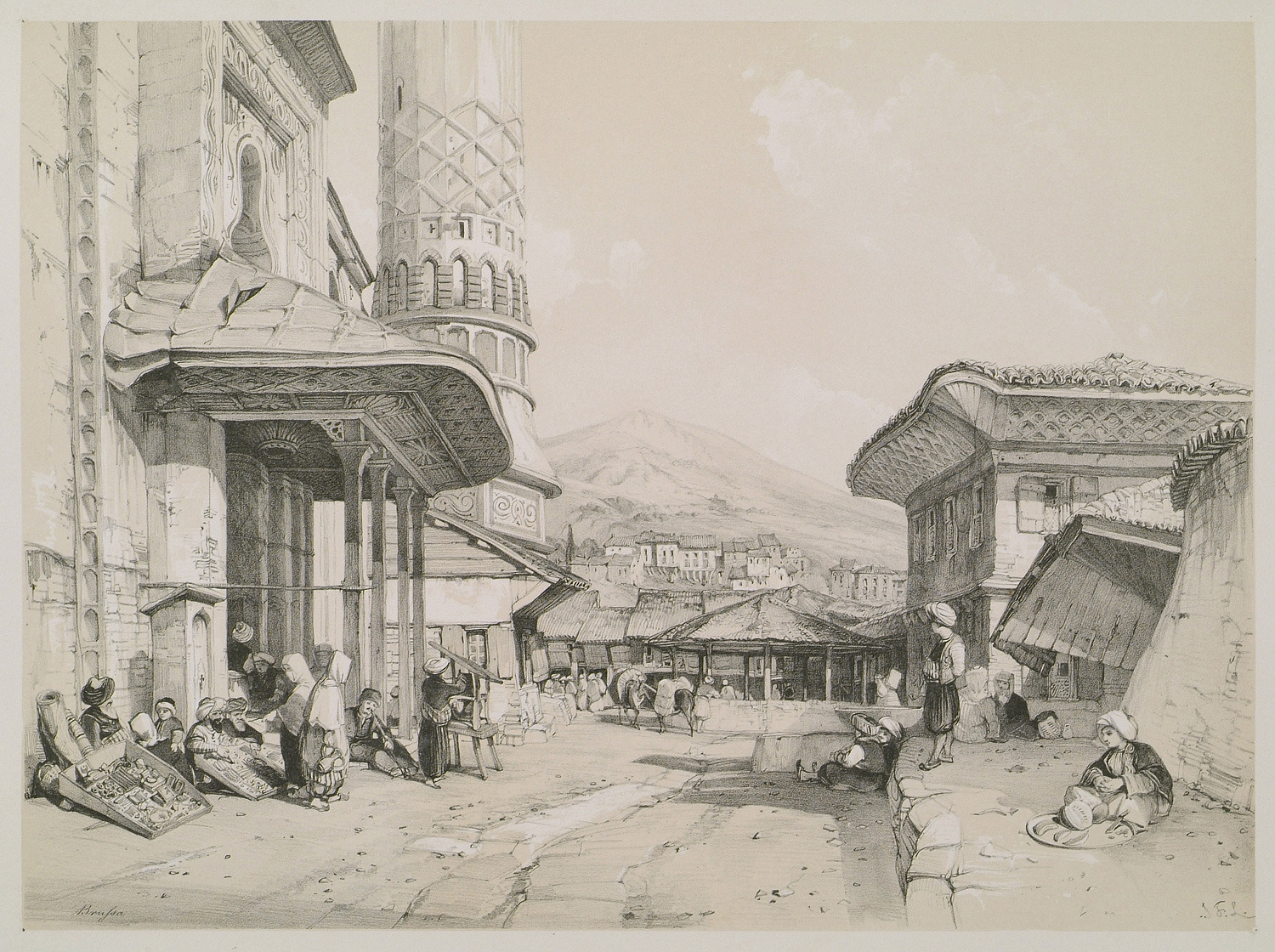This detailed pencil sketch depicts a bustling street scene in an ancient city in black and white. Dominating the left side is a large stone building with an awning, under which several people, including a vendor with a tray, are seated on the ground. Adjacent to this building stands a tall, cylindrical tower that extends beyond the frame. On the right side of the street, a shorter, two-story building is visible. Along the pathway, people wearing traditional, possibly ancient attire, including turbans, are engaged in various activities such as sitting, standing, and conducting business. Some appear to be selling goods. Midway down the street, there are animals carrying loads on their backs. The scene is set against a backdrop of smaller houses and a prominent hill or mountain under a clear sky with a few white clouds.